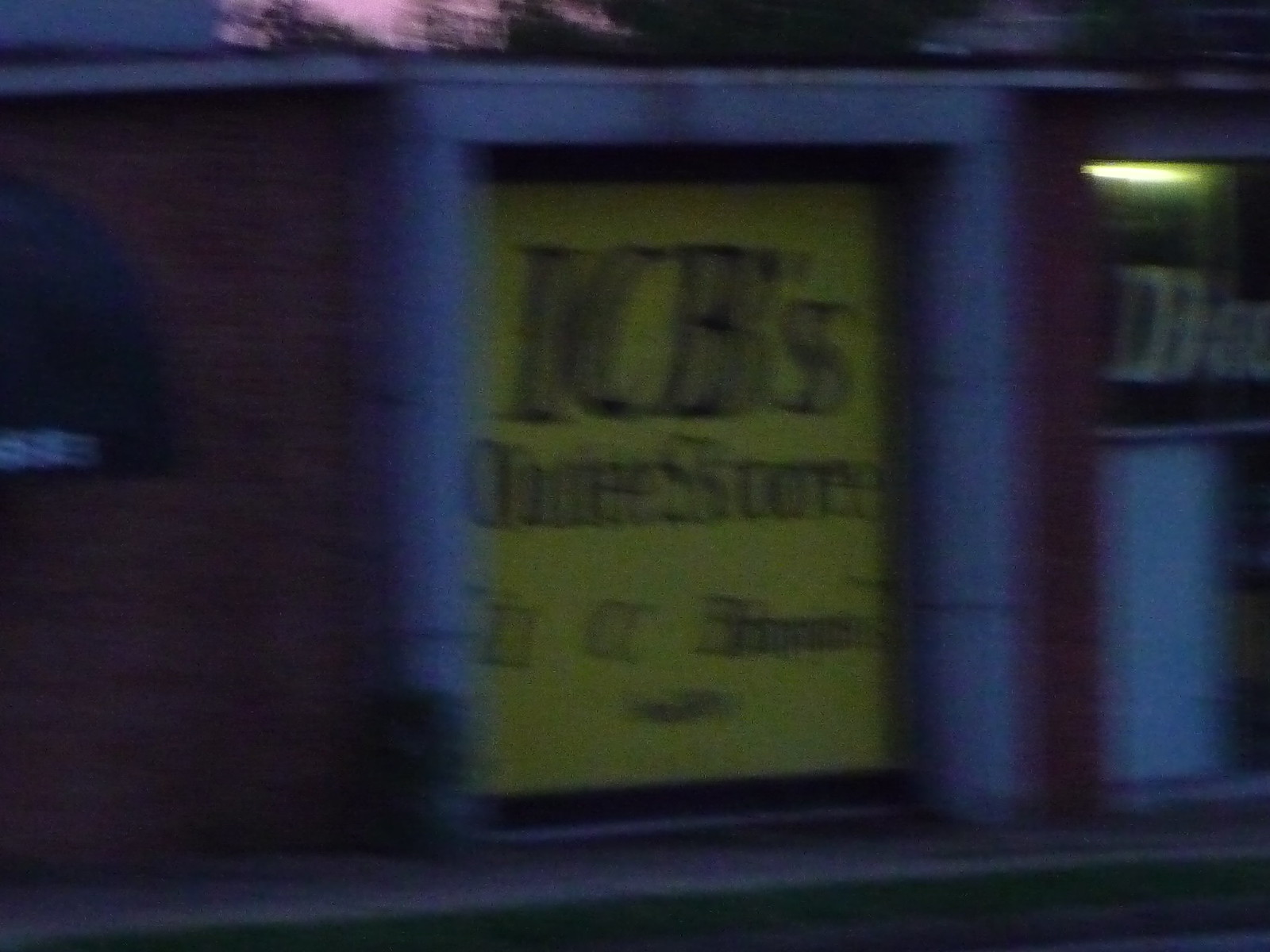The image depicts a blurry, dark scene with a yellow sign featuring black lettering that reads "ICB's something store." The sign is possibly part of a storefront and is outlined with a blue edge. The surrounding area has a mix of textures and colors, including a maroon or red to dark brown brick wall. A light glows inside a window, suggesting an interior space, while a D and possibly other characters are faintly visible on the window and nearby in white text. The upper portion of the image shows a pinkish hue in the sky, likely indicating sunset, with silhouettes of trees visible. The overall exposure is low, contributing to the difficulty in deciphering more details.